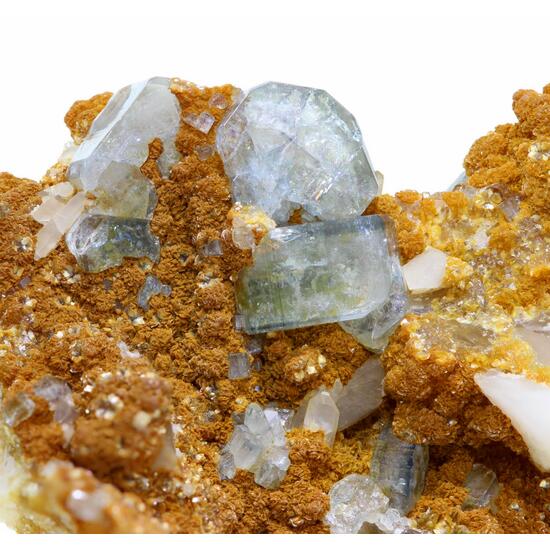The photograph captures an indoor setting with a pristine white background, showcasing an arrangement of translucent silver or white crystals, potentially quartz. There are about five to six crystals, including two prominent ones in the middle; one shaped like a small rock and another resembling a slightly rectangular form. These misty, glass-like crystals, some with hints of blue or grey, rest atop a bed of brownish-orange elements, which could be either a powdery substance, brown sugar, or dirt, giving a naturalistic appearance. Scattered throughout, this brown material adds texture and contrast to the clear stones. The bottom left corner features a slightly out-of-focus green element, adding an additional layer of color to the composition. The image is devoid of text or human presence, focusing solely on the intricate interplay between the crystals and the surrounding material.